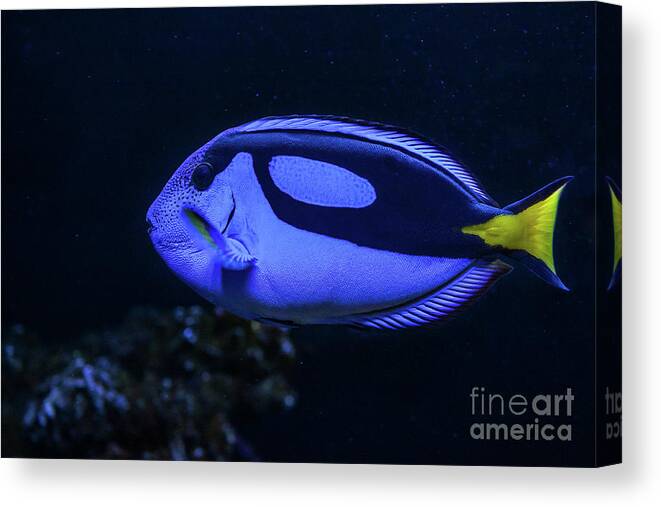The image depicts a detailed, colorful canvas print of Dory, the blue fish character from "Finding Dory." This artwork showcases the fish's distinctive features: a primarily blue body with a long black stripe extending from its eye to the back, encompassing the tail except for a vivid yellow triangular section. Dory's fins are short and blue, curving backward towards the tail. The canvas has a 3D appearance as it wraps around a rectangular frame, and the right side shows a reflection of the tail. On the bottom right, there is a watermark that reads "Fine Art America." The background is predominantly black, with a rocky area on the bottom left highlighted in blue accents, giving depth to the underwater scene.